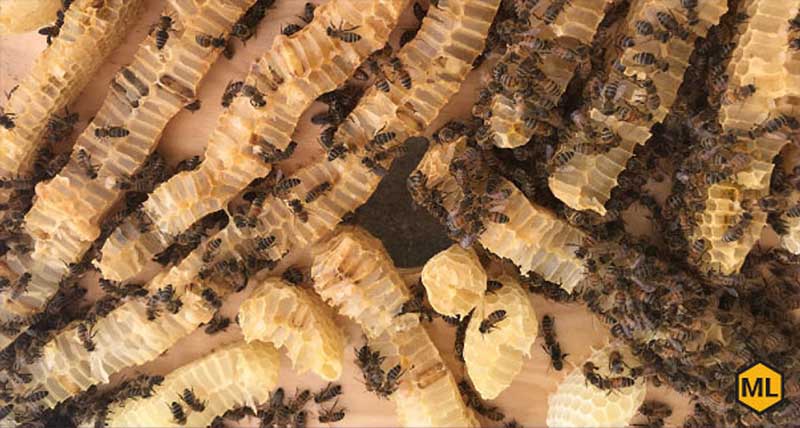This vivid, close-up color photograph provides a first-person perspective as if looking straight down into a hive teeming with life. The image reveals a complex structure of honeycomb strands arranged vertically and horizontally against a pinkish background. Each strand is bustling with brownish bees, showcasing their black-banded abdomens and clear wings. The bees are predominantly clustered in the bottom right and upper right portions of the hive, though they are spread throughout with their numbers likely in the thousands. 

A bold yellow hexagon logo with the letters 'ML' in black is positioned in the lower right corner, adding a striking visual element to the intricate natural scene. The hive's myriad compartments, disrupted and partially exposed, reveal the organized yet chaotic life within this thriving colony.